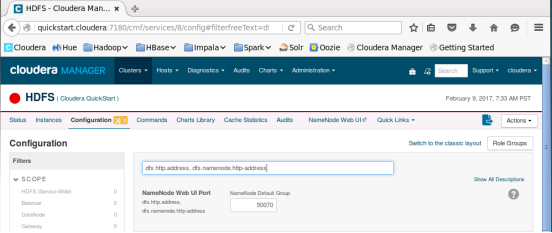This is a detailed screenshot of a desktop interface featuring the Cloudera Manager. At the top, there is a single open browser tab labeled "C logo, HDFS-CLOUDERA..." with a close button (X) beside it, and a plus sign to open a new tab. The rest of the tab bar is light gray. 

Below the tab bar, the address bar contains a left arrow (back button), followed by the URL "QUICKSTART.CLOUDERA" and additional site-specific path. Next to it are a refresh icon, a search box, and a save icon, alongside other miscellaneous icons, including a menu button represented by three horizontal lines.

The bookmarks toolbar below the address bar includes several bookmarks: "CLOUDERA", "HUE", "HARDPOP", "HBASE", "IMPALA", "SPARK", "SOLR", "OOZIE", "CLOUDERA MANAGER", and "GETTING STARTED".

The main content area begins with a blue banner featuring the word "CLOUDERA" in white letters and "MANAGER" in blue letters. Below the banner, there's a navigation menu with drop-down options for "CAREERS", "HOSTS", "DIAGNOSTICS", "AUDITS", "CHARTS", and "ADMINISTRATION".

In the central part of the page, under the section titled "HDFS-CLOUDERA QUICKSTART," there are multiple menus. The left sidebar displays options for "CONFIGURATION".

The main section of the page has a gray box containing a white search box with a blue outline, and various text along with another input box.